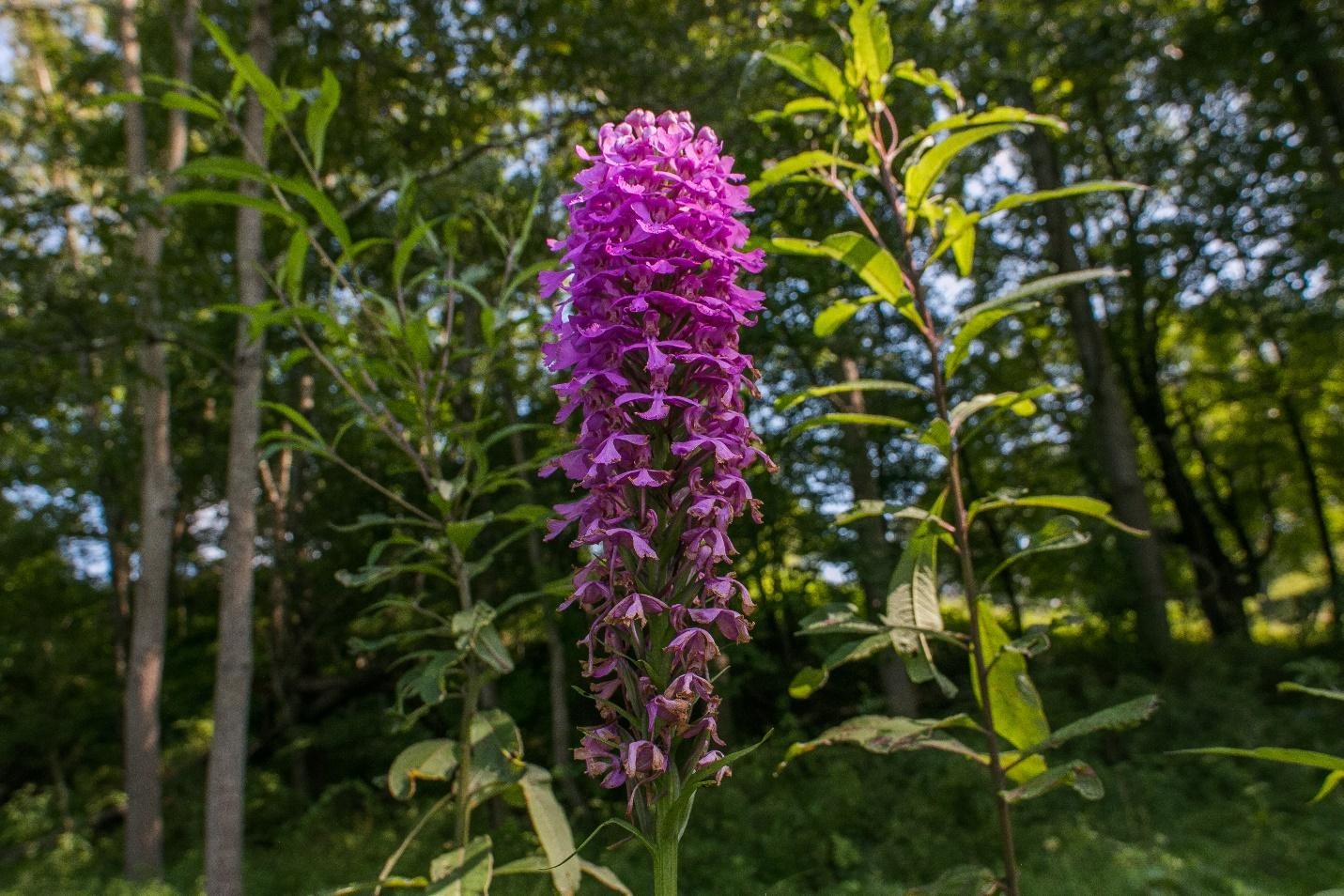This photograph captures a close-up of a striking, bright purple flower that dominates the center of the frame, extending almost the entire height. The flower, reminiscent of a pinecone in shape but vividly purple, features numerous small, bell-shaped or angel-shaped pink blossoms hanging down, possibly numbering in the dozens or even a hundred. It has a green stem with thin leaves extending from it, some of which show signs of having been chewed.

Flanking the main flower are two slender offshoots with green leaves, adding to the natural complexity of the scene. The background is slightly blurred but reveals a mix of plant life, including a lush, green leafy plant on the left and a drier, somewhat withered one on the right. Further back, a forest scene emerges with spindly, pale-trunked trees reaching up to a green canopy, all somewhat obscured to focus attention on the flower. Flecks of blue and white sky peek through the foliage, adding depth to this vibrant nature scene.